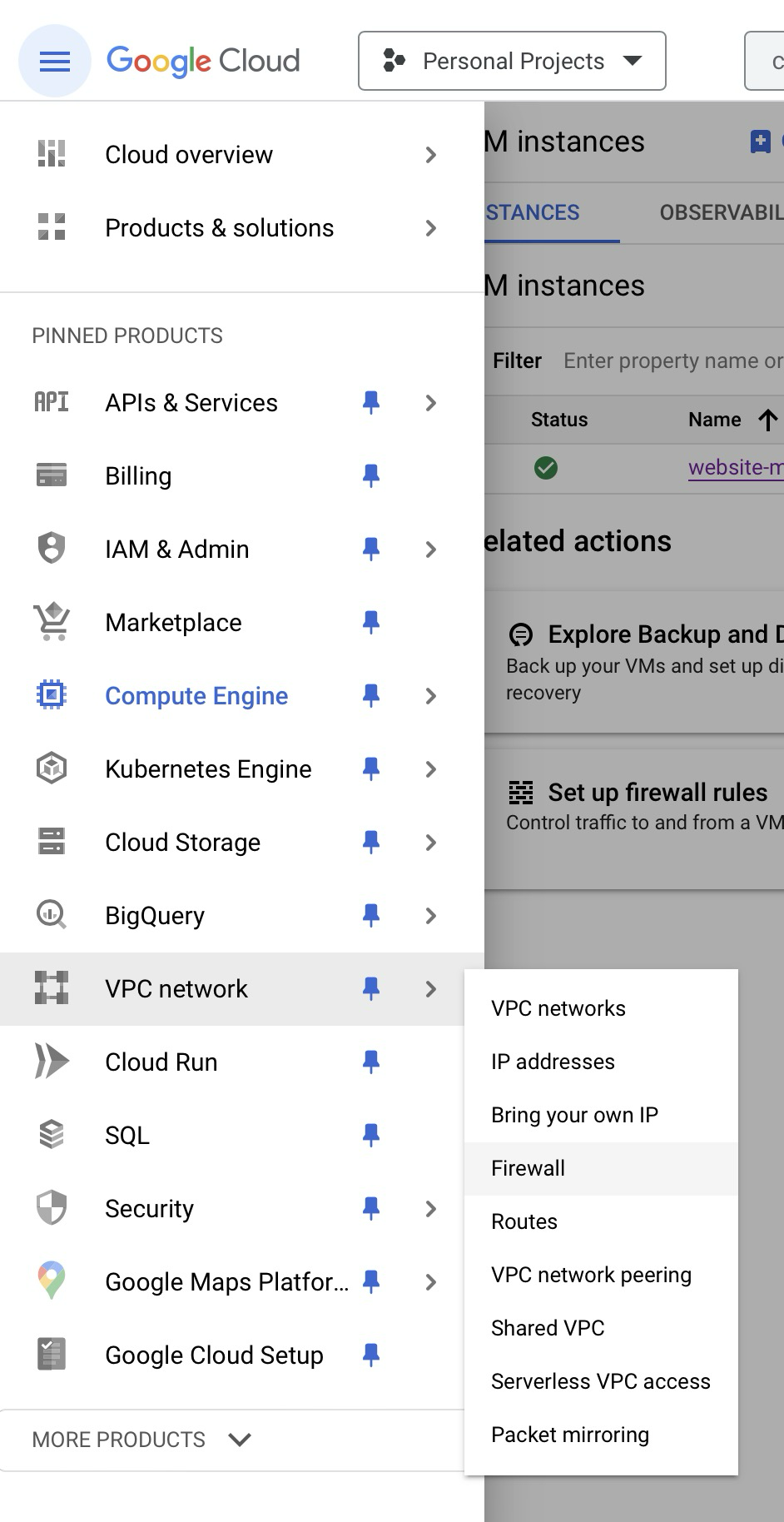The image features a Google Cloud interface. At the top, the header displays "Google Cloud" prominently, accompanied by several bars. To the right of this, there is a label titled "Personal Projects" with a dropdown tab. Below the header is an extensive row of tabs labeled: Cloud Overview, Product and Solutions, API and Services, Billing, IAM and Admin, Marketplace, Compute Engine, Kubernetes Engine, Cloud Storage, BigQuery, VPC Network, Cloud Run, SQL, Security, Google Maps Platform, Google Cloud Setup, and More Products.

Each tab is marked with distinctive icons to its left—ranging from a credit card for billing to a shield for security. Icons also include a computer chip, a shopping cart, hard drives, a magnifying glass, interconnected boxes, stacked boxes, a shield emblem, a pin, and a box with a checkmark.

Adjacent to the tabs, a blue pin symbol can be seen to the right of several entries, along with arrows indicating further options. The interface elements are overlaid against a background image of a main street, adding contextual depth. To the right, various text boxes provide additional instructions, such as "Set Up Firewall Rules," guiding users through potential configurations and settings.